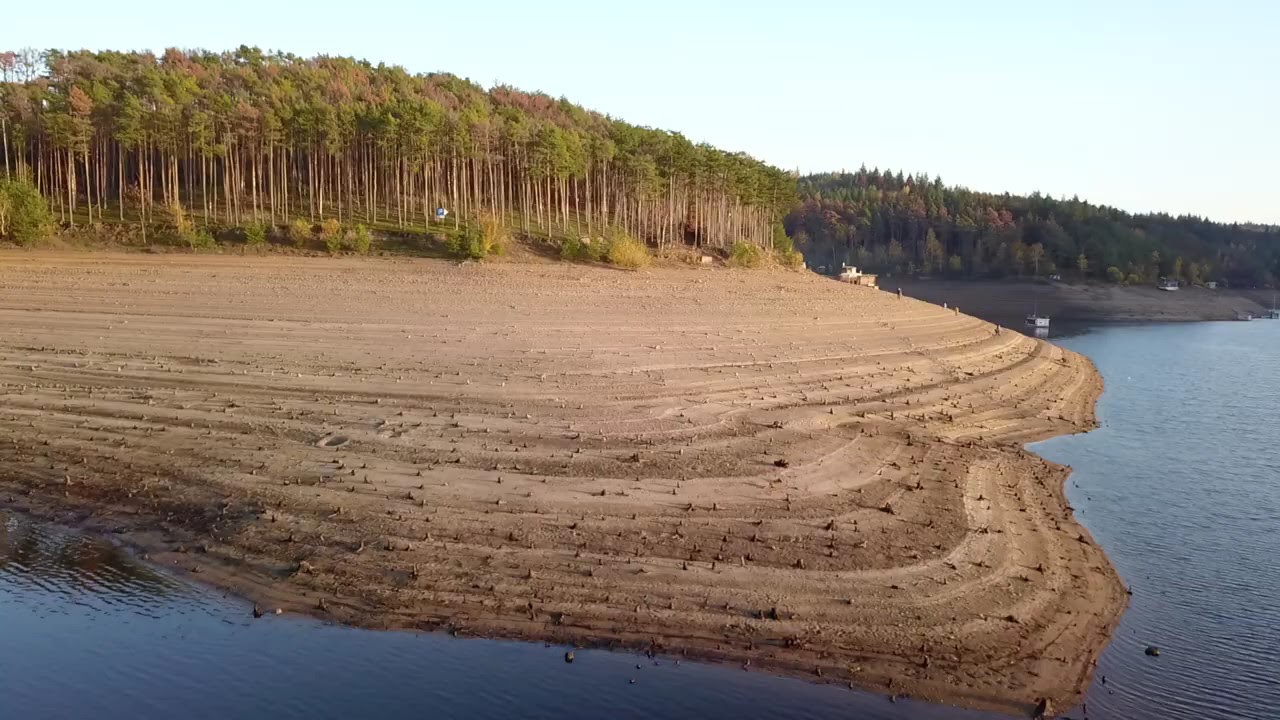This photograph captures a daytime scene of a drought-stricken lake with a significant receding water line, revealing approximately 200 feet of dry, tan shore that transitions to a darker tan closer to the water. The lake is framed by tall, barren trees with green and brown foliage concentrated at their tops, situated on a hill above the exposed lakebed. The sandy shore appears layered, with small dark spots that could either be brown birds or plant stems, scattered across the ground. In the distance, a large boat is visible on the upper left corner of the image, along with a buoy on the water. People are seen standing on the revealed shore, some engaged in fishing, while a smaller boat floats near the dip between what looks like two side-by-side islands.